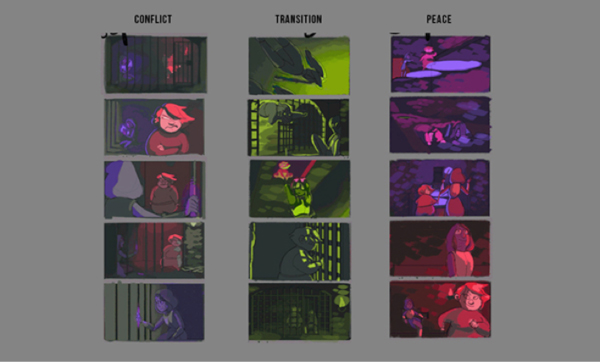The image displays a gray background with three vertical columns of five cartoonish pictures each, titled "Conflict," "Transition," and "Peace" in black text at the top of each respective column. The "Conflict" column depicts a series of scenes involving black stripes, resembling jail bars, and characters in distress—one blue and one red. These characters are seen moving through various emotionally intense scenarios, including one where only the red character is visible, surrounded by bars. The "Transition" column, characterized by dominant lime green and black colors, seems to illustrate a journey towards liberation, with fewer restraining bars and a more dynamic interaction between characters, suggesting a move away from confinement. The "Peace" column, in shades of purple and red, portrays serene and harmonious scenes with one or two characters in each image, absent of any jail bars, evoking a sense of resolution and calm.